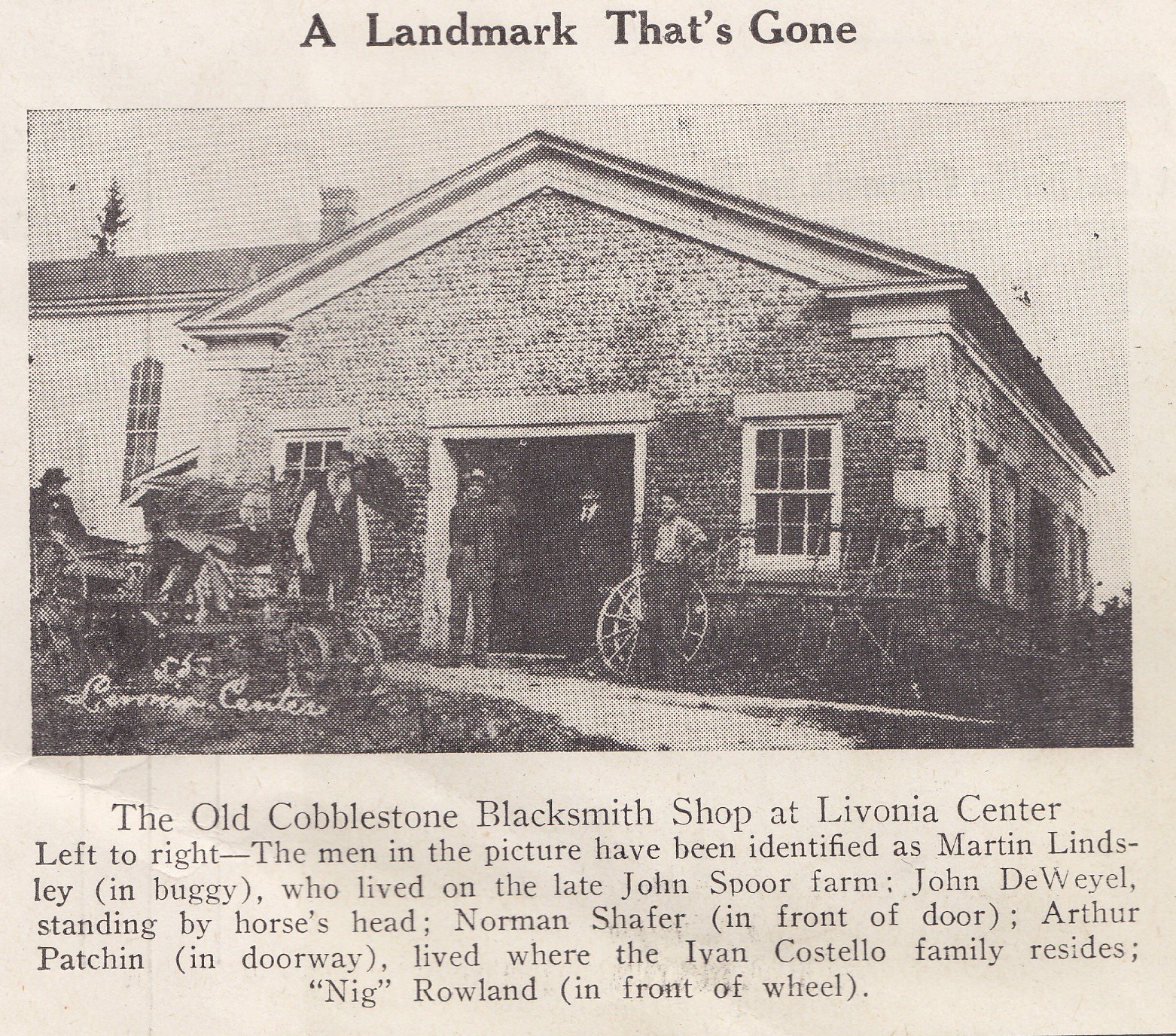An old black and white newspaper clipping titled "A Landmark That's Gone" showcases a photograph of the Old Cobblestone Blacksmith Shop at Livonia Center, England. The brick building, appearing fairly aged, features two front windows and a large front door with a shaped roof. In the scene, several men are positioned in front of the building: Martin Lindsay sits in a buggy by the horse on the left, John Deweel stands by the horse's head, Norman Schaefer is in front of the door, Arthur Patchen stands in the doorway, and Nig Rowland is in front of the wheel. A secondary building is visible behind them, along with the sky and the top of a tree emerging from behind the roof on the left. A small patch of shrubbery appears in the lower right background. The photograph, likely taken in the late 1800s or early 1900s, captures a historic moment in the once-busy blacksmith shop now long gone.